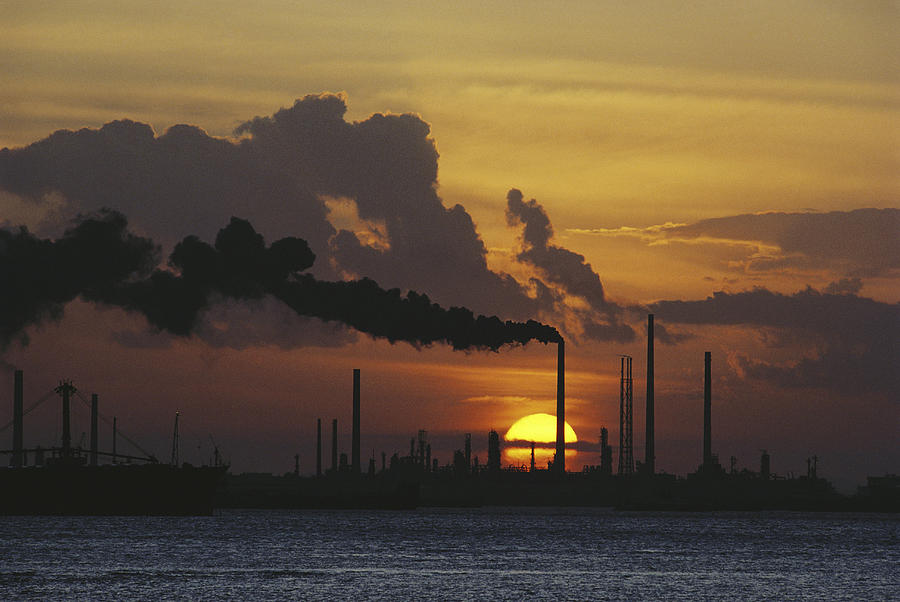The image captures the serene yet industrial scene of a sunset over a water body, possibly a bay, lake, or river. The sky is a stunning mix of yellow, orange, pink, and red hues, embellished with dark gray clouds. The sun, almost set, is a bright yellow orb resting just above the horizon. In the foreground, dark blue waters ripple, suggesting a breezy evening.

Dominating the middle of the image is a city skyline silhouetted against the vibrant sky, featuring several smokestacks of a large industrial facility, likely a foundry or power plant. The tallest smokestack, positioned centrally, emits thick black smoke that billows leftward, casting a dramatic shadow over the scene. Smaller smokestacks, although visible, remain inactive. To the far left, a large barge or sailing vessel floats, also in silhouette, adding to the depth and complexity of the scene. The interplay of natural beauty and industrial elements creates a poignant juxtaposition, capturing both the serenity of the sunset and the imposing presence of human industry.